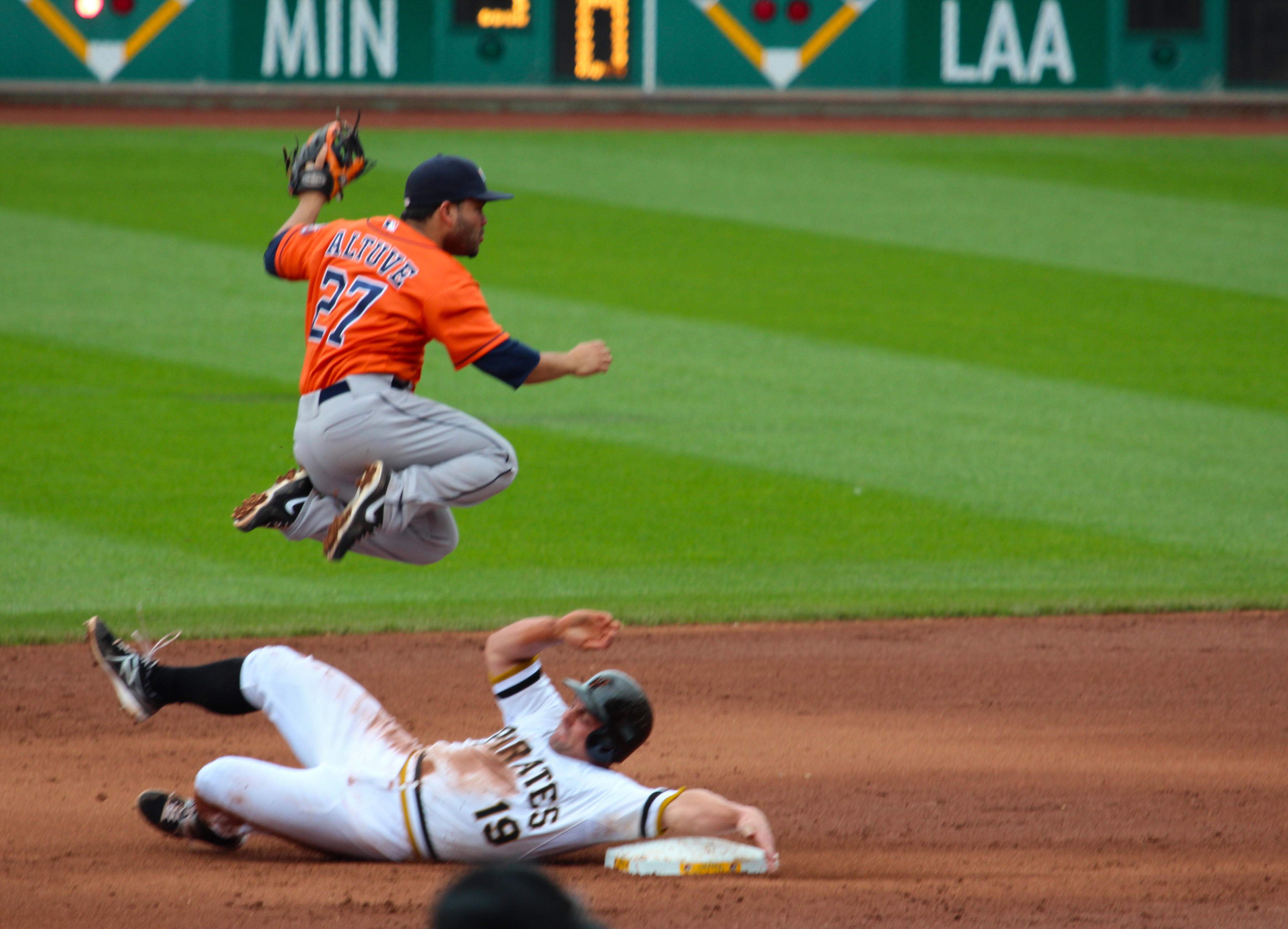In this dynamic photograph taken at a baseball game, two players are captured in the midst of a dramatic play on a baseball diamond. The player in white, sporting a jersey that reads "Pirates" in black font with the number 19, is wearing a black helmet and sliding hand-first past a base, his fingers just grazing the bag. Meanwhile, the opposing player in an orange jersey with "L2" and "27" in blue font, gray pants, baseball gloves, and a blue cap, is caught mid-air, jumping over the sliding player. They are both on the dirt part of the baseball field, and a bit of the outfield is visible in the background. Interestingly, the outfield appears to double as a soccer field, evidenced by the distinct light and dark green stripes and a low wall visible in the upper portion of the image. The border area of the field features a green-colored board with logos and banners in yellow and red and digital numbers showing scores, with text elements like "MIN" and "LAA" making an appearance.